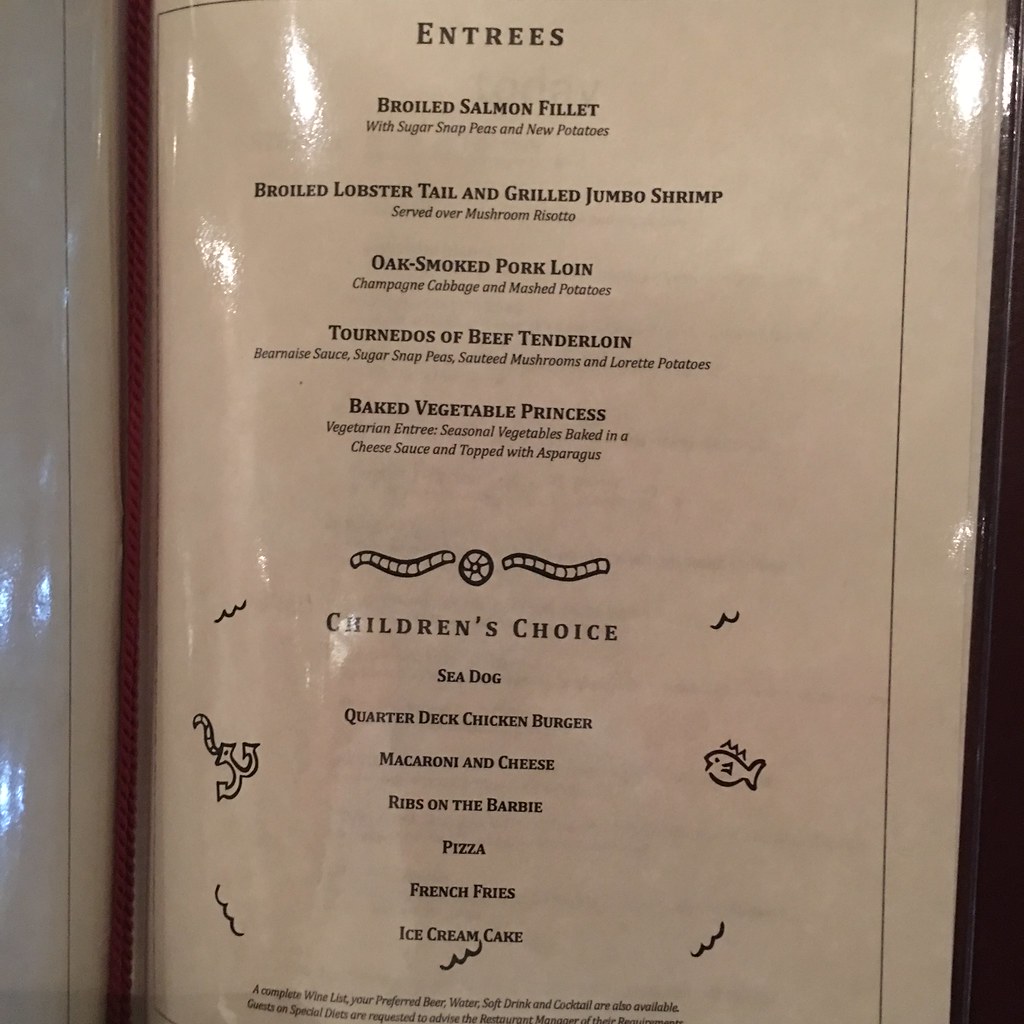A white page bordered by a thin black line, possibly part of a restaurant menu, is encased in a protective clear plastic covering. The page is titled "Entrees" and lists a variety of mouthwatering dishes. The offerings include broiled salmon fillet served with sugar snap peas and an unidentified potato dish, broiled lobster tail paired with grilled jumbo shrimp atop mushroom risotto, and oak-smoked pork loin accompanied by champagne cabbage and mashed potatoes. Another option is beef tenderloin tournedos draped in béarnaise sauce, served with sugar snap peas, sautéed mushrooms, and yet another type of potatoes. Additionally, a vegetarian entree named "Baked Vegetable Princess" features seasoned vegetables baked in a cheese sauce, topped with asparagus.

At the bottom of the page, a section labeled "Children's Choice" is decorated with nautical-themed doodles—a small anchor on the left and a little fish on the right. This section lists kid-friendly options including a seadog, quarter-deck chicken burger, macaroni and cheese, ribs on the barbie, pizza, french fries, and ice cream cake. There is no other text or indication of the restaurant's name.